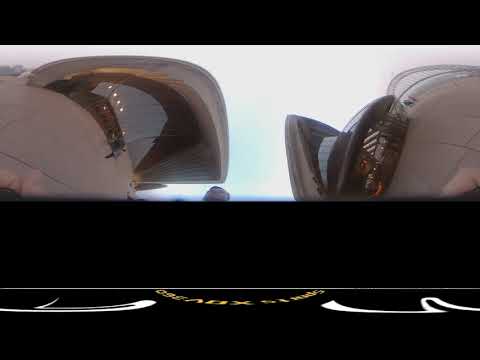The image is a confusing, photorealistic scene that appears to be rotated 90 degrees from its normal orientation. In the top half, there are two light gray or white structures that seem to be buildings. These buildings have white paneling and windows, with one structure on the left having a curved, C-shaped roof or ceiling. The windows are oriented in a way that suggests the buildings might be seen from an unusual angle. The background depicts what could be a suspension bridge and a sky that ranges from blue to gray with white clouds.

The bottom half of the image is completely black except for the bottom quarter, which has a stretched design, possibly a logo, in bright yellow and white. There are indistinct swirls of white on either side and illegible text below a white line. The ground beneath the buildings is a light brown color, and due to the poor resolution, it is challenging to make out additional details. The overall impression is of a highly disorienting and abstract scene with elements of urban architecture juxtaposed against a seemingly natural background.